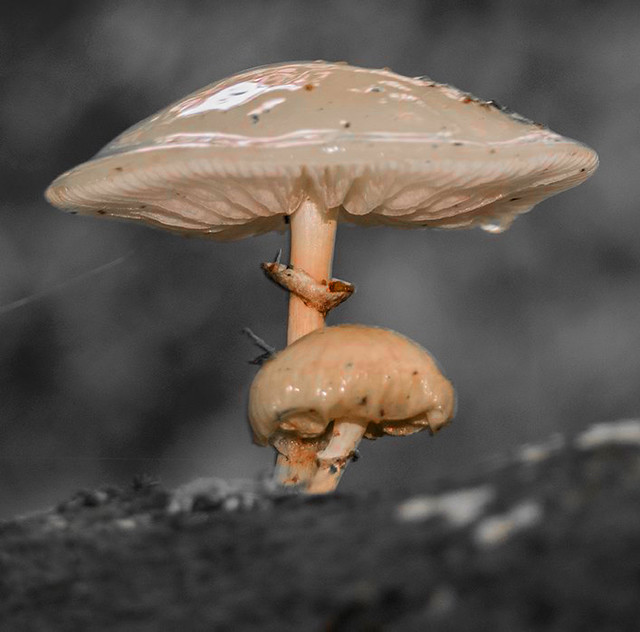This close-up outdoor photograph showcases two mushrooms positioned on a dark, slightly blurred wooden log. The background transitions through various shades of gray, from cloudy white to almost black, further emphasizing the natural texture of the scene. The prominent mushroom dominates the upper portion of the image, characterized by its glossy, white cap adorned with fine black specks that give it a polka-dotted appearance. The cap's shiny, moist surface reflects the ambient light, accentuating its smooth texture. Below the cap, the underside resembles intricately folded paper, leading down to a stalk that transitions from white to a light peach or brown hue. Attached to this stalk is an indistinguishable object that could be part of the mushroom or possibly a small bug. Positioned at about a third of the height of the larger mushroom, a smaller mushroom mimics the same aesthetic features, including the glossy cap and speckled surface. The ground beneath the mushrooms merges into the background with dark gray and white smudges, completing the delicate and detailed composition of this intriguing natural scene.